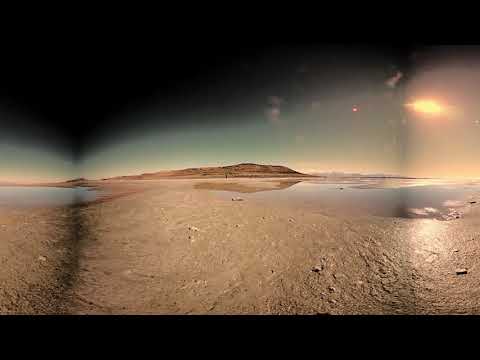This photograph captures a desolate desert landscape, likely depicting a dried-up lakebed during a drought season. The ground, primarily light tan with cracks, stretches out toward a shallow, reflective pool of water. The reflection reveals a small mountain in the far distance. The sun, casting a golden glow, sits near the horizon on the right, suggesting either sunrise or sunset and painting the sky in hues of blue, yellow, and orange. The image, low in resolution, shows an outdoor scene with no greenery, emphasizing the barren environment. A partially closed lens causes black borders at the top and bottom, adding to the photo's stark and rugged feel. The dark, underexposed area on the left side further contributes to the photo's dramatic contrast.